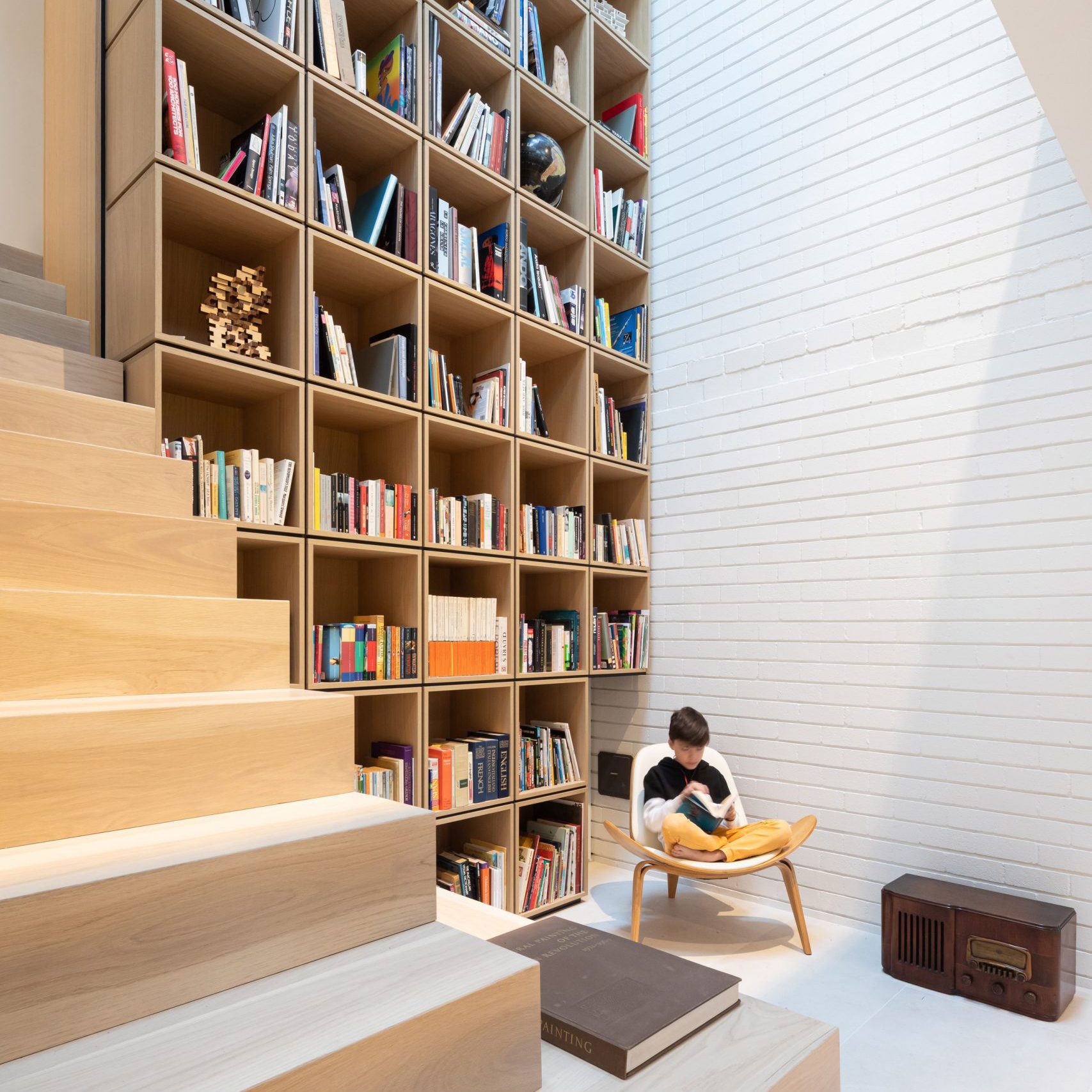In this photorealistic image, a young boy is seated cross-legged in a modernist, curved wooden chair with three legs, reading a book. He is positioned near the bottom center of the photograph, adjacent to a white-painted brick wall that rises magnificently to an estimated height of 25 to 30 feet, indicating a space with exceptionally high ceilings. The room exudes a minimalist, contemporary vibe, emphasized by a strikingly designed bookshelf made up of cubes stacked together. This bookshelf, filled with a variety of hardcover and softcover books along with some artistic items and a globe, commands attention with its towering presence, featuring eight rows of cubical shelves that reach an impressive height of about 25 to 30 feet. 

To the left of the image, there's a similarly modern staircase with no railing, composed of light color wood that blends harmoniously with the minimalist aesthetic. Sunlight from above illuminates the scene, enhancing the serene ambiance of the space. Across from the chair, a dark brown radio adds a touch of retro charm to the setting, and a secondary book is placed in the foreground. The overall scene could depict an interior of either a house or a library, blending sophistication with a cozy, reading-friendly atmosphere.